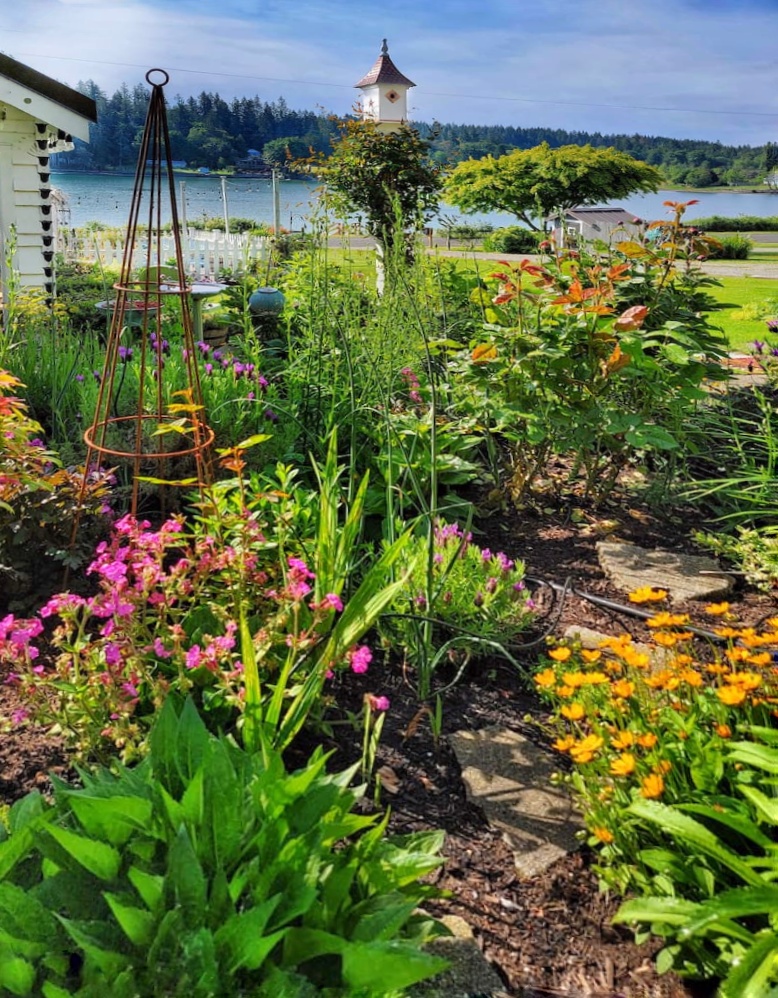This daytime photo, likely taken in spring, captures a detailed view of a flower garden adjacent to a small white cottage with a black roof and white eaves. The garden, composed of various plants with vibrant pink, orange, yellow, and green foliage, is adorned with a rock pathway winding through it. A metal tower, designed for climbing plants, is situated among the flora. Central to the garden is a birdhouse, adding a quaint touch. The scene transitions to a lush green lawn leading to a serene lakefront. In the background, a white tower with a brown peaked roof stands tall near a large tree, and beyond the lake, a dense forest of mixed evergreens and possibly Japanese maple trees is visible under a blue sky dotted with white clouds.